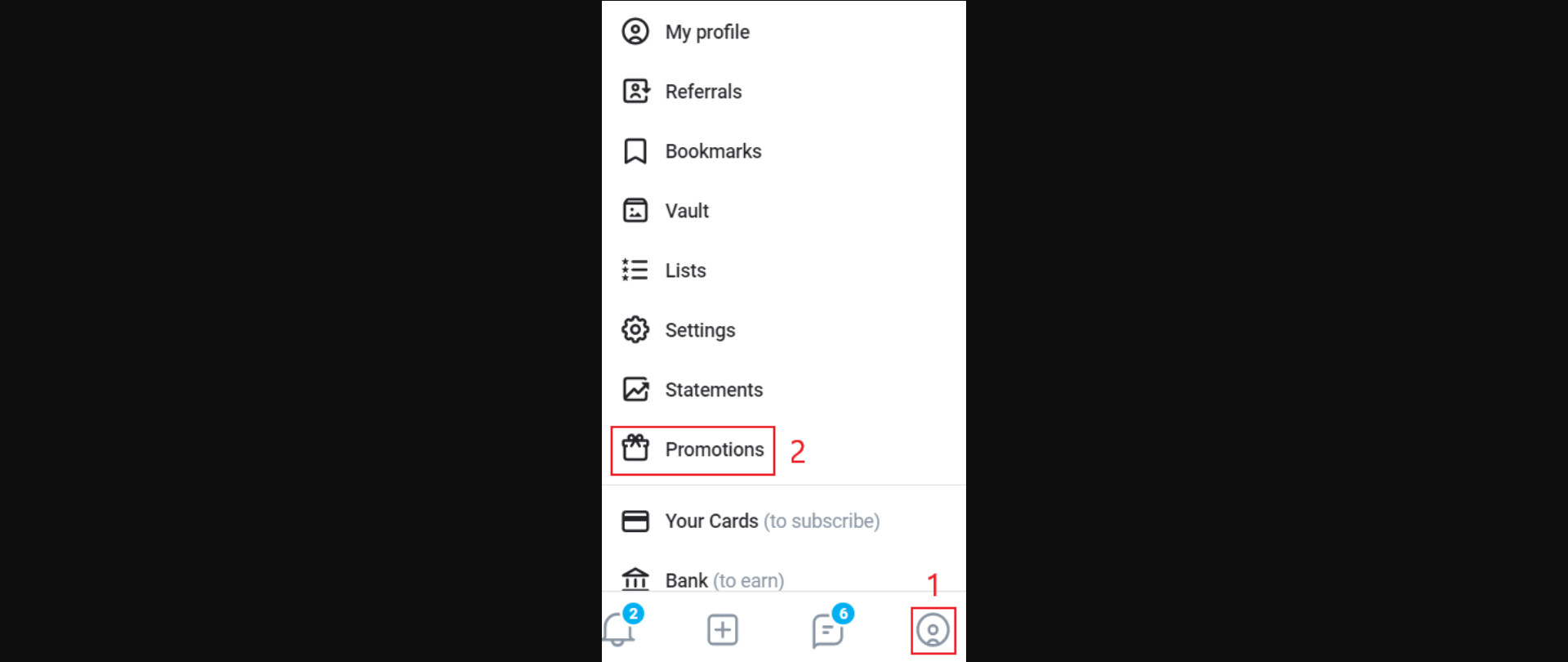The image showcases a phone profile page with a clean, white interface and black text set against a black rectangular background. At the top, "My Profile" is listed in black font accompanied by a small person icon on the left. Below it are several items:

1. **Referrals**: Features a small person icon and a square icon.
2. **Bookmarks**: Displayed with a frequently used bookmark icon on the left.
3. **Bolt**: Marked by a lightning bolt icon.
4. **List**: Represented by a list icon.
5. **Settings**: Denoted by the classic gear icon.
6. **Statements**: Has an icon resembling a bar graph with an arrow pointing upward to the right.
7. **Promotions**: Highlighted with a gift box icon, encircled by a red rectangular outline with a red notification badge indicating the number "2".
8. **Your Cards**: Labeled with a card icon on the left, followed by "to subscribe" in gray font.
9. **Bank**: Shows a bank icon and "to earn" in light gray parentheses.

At the bottom is an area with additional icons:

- A timer icon with the number "2" in blue, accompanied by a plus sign.
- A text symbol with a blue circle and the number "6".
- A unique circular icon with a smaller circle in the middle and a half-moon shape at the bottom, outlined in red, with a red notification badge marked with the number "1".

This page meticulously organizes profile-related options and functionalities, making them easily accessible and visually distinguishable by their respective icons.